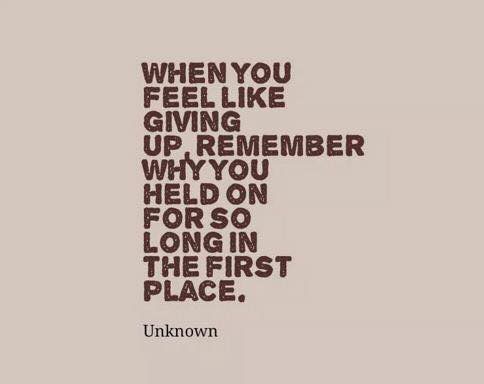The image is a square, likely saved from the internet due to noticeable JPEG artifacting, with a plain, light brown (beige) background. Prominently centered is a grungy, dark brown text with a rough, aged look, written in all caps, that reads: "When you feel like giving up, remember why you held on for so long in the first place." Below this, in a simple, plain black Arial font, is the attribution "unknown." The overall aesthetic suggests it’s a digitally created graphic, often seen on social media platforms like Facebook or Instagram. The background and text together create a vintage, slightly pixelated appearance, enhancing its rustic feel.